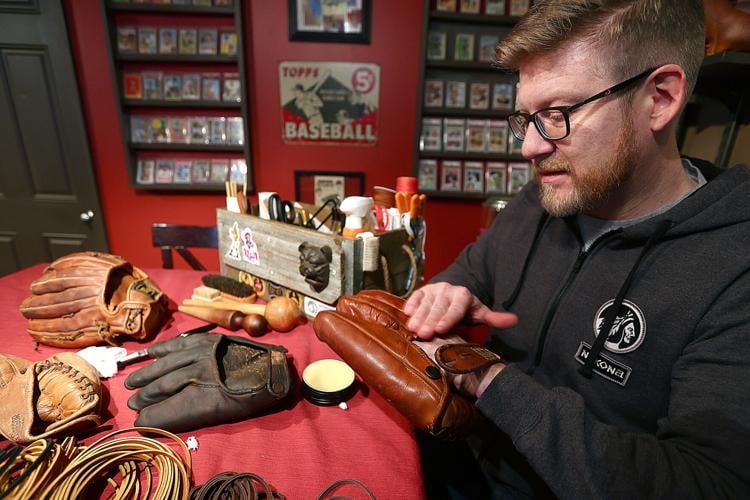In this image, a middle-aged Caucasian man with short brown hair and dark-framed glasses is seen working on a baseball glove. He has a reddish-brown beard with specks of gray and wears a dark gray hooded sweatshirt featuring an embroidery of a Native American with a headdress, likely the Redskins logo. Underneath, he has on a gray shirt. The man is intently examining a dark brown leather baseball glove with his right hand inside it and his left hand adjusting it.

He is seated at a table covered with a red tablecloth, protecting the surface, on which several other baseball gloves are displayed. These include a light brown glove with some fading, a tan-colored glove, and another chocolate brown glove. Surrounding the gloves are various leatherworking tools, coiled straps of leather in different shades, and what appears to be a cream or saddle soap for polishing the mitts.

The background reveals a setting richly adorned with baseball memorabilia, suggesting it could be a museum, a store, or his private collection. The walls are painted a deep red, complementing dark, almost black shelves filled with baseball cards encased in protective holders, as well as various posters and frames, including one prominent poster with the words "Topps 5-Cent Baseball" and an image of a person swinging a bat. A dark gray door is visible to the side, closed, adding to the room’s enclosed, focused atmosphere.